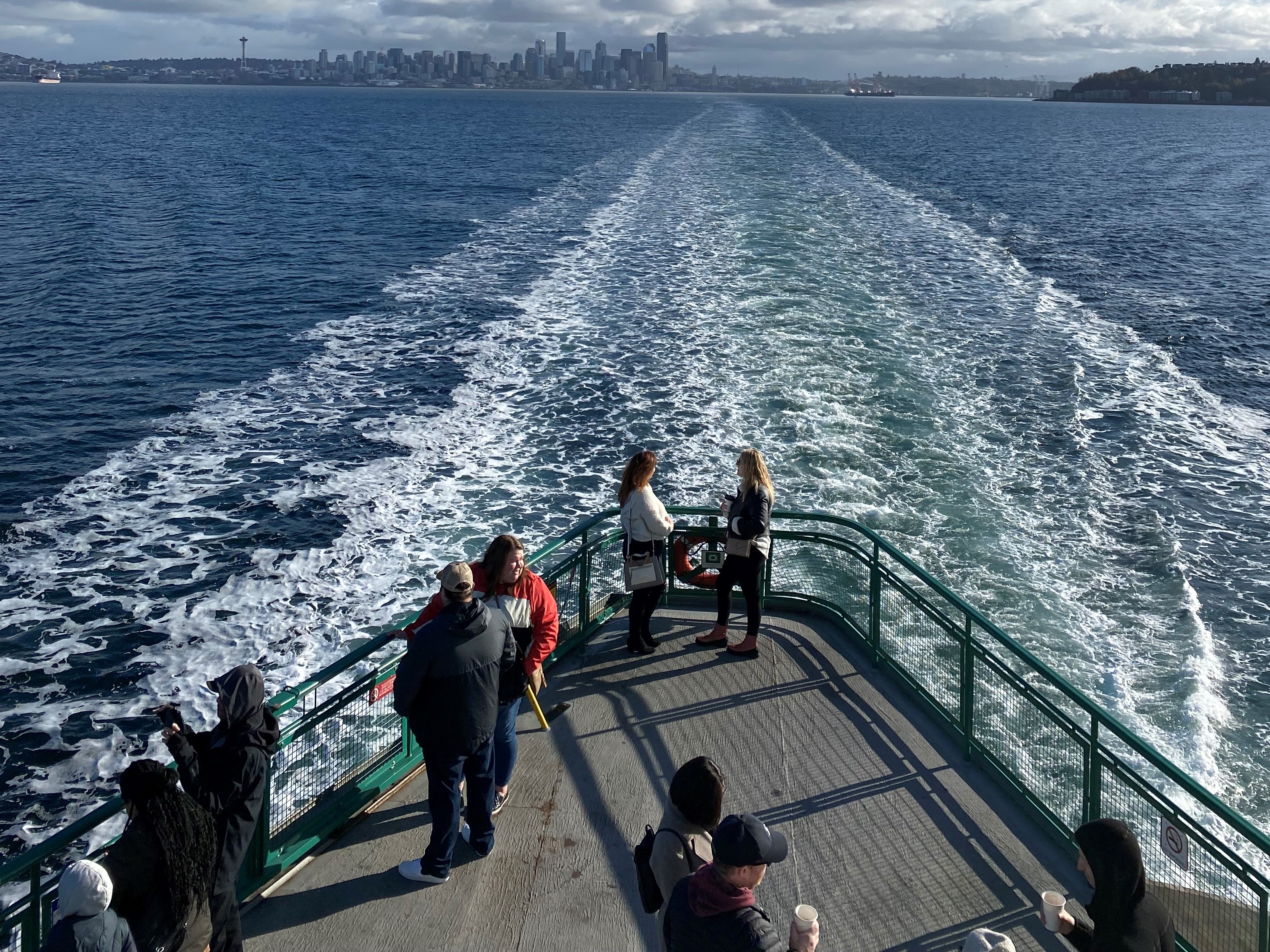This image captures a candid moment aboard a large passenger ship, likely a ferry traveling through a river or lake near a major city. The photograph is taken from the second floor of the vessel, focusing on the back end where various people are scattered. The railings, painted green and reaching chest height, frame the scene. 

Around nine individuals are visible: three in the bottom left corner, bundled in coats and gazing off to the left; two more situated closer to the boat's edge, including a man and a woman observing their surroundings; and another small group of three in the bottom right, casually holding drinks that appear to be coffee and engaging in conversation. Some people are also seen taking pictures or simply enjoying the view.

In the background, a hazy city skyline punctuated by skyscrapers stretches across the horizon, possibly indicating a city like Seattle, San Diego, or New York. The distinctive architectural silhouettes, potentially including landmarks like the Space Needle, suggest urban density far off in the distance. A couple of other boats can barely be made out, indicating moderate water traffic. The wake generated by the ship creates sea foam and waves behind them, adding a dynamic element to the serene atmosphere as the vessel moves towards its destination.